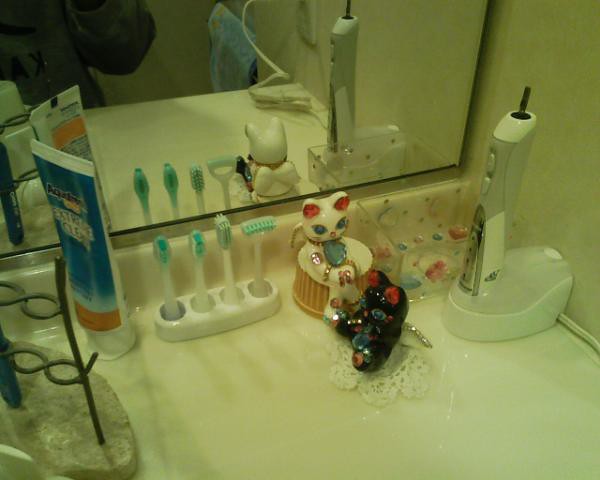The image appears to be taken from the early 2000s and depicts a section of a bathroom countertop with a large, frameless wall-mounted mirror. The setup includes a variety of toiletries and personal items. In the middle, there's an upright Aquafresh toothpaste tube alongside a rack featuring four different types of electric toothbrush bristles. Positioned on the right is an electric toothbrush charging station, with the toothbrush base resting on it, but without a brush head attached. 

Adjacent to this setup is a clear acrylic box, possibly containing nail care items or other personal effects. The scene also features a black Maneki-neko (lucky cat) figurine, which is actually a trinket box with pink ears, blue eyes, and a blue jewel on its chest. Sitting on a small white doily next to the cat figure is a porcelain mini bear lying on its back. There is another holder present which appears to possibly store manual toothbrushes, adding further to the eclectic assortment of items on the countertop.